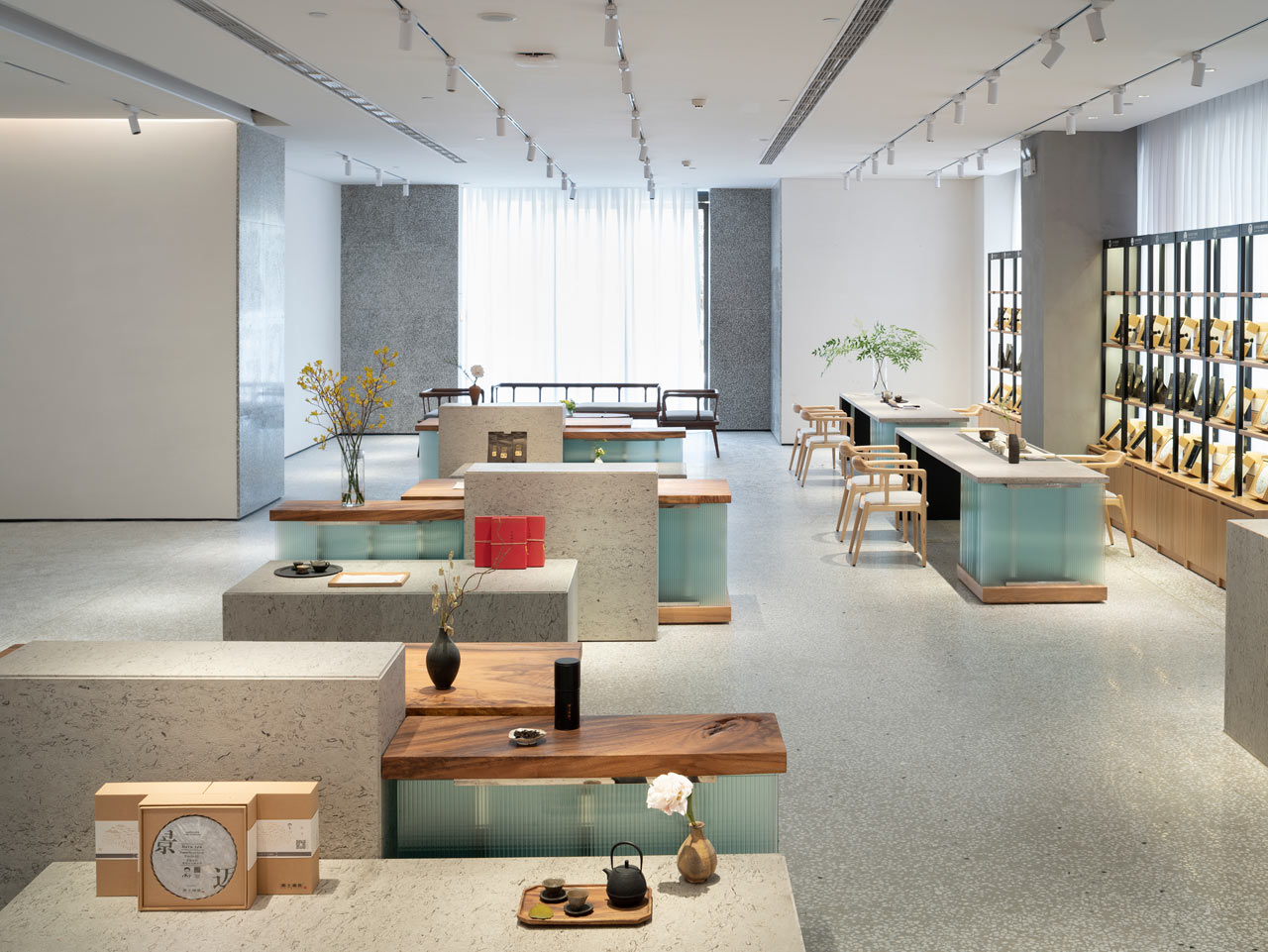The image depicts the interior of a Japanese-style restaurant, adorned with various detailed elements. In the foreground, there's a small desk area featuring a black teapot set placed on a wooden base, flanked by a vase containing a delicate white flower on the right and three boxes on the left. Surrounding this setup, the scene reveals several wooden tables and chairs with white cushions, contributing to the inviting atmosphere. The tables are thoughtfully embellished with tea kettles and small flower arrangements. Behind these tables, black shelves with brown wooden accents house yellow objects, adding a subtle contrast to the decor. On the left, there's a white marble-like bench, juxtaposed with a green texture below. The floor extends to the back of the room where a prominent window allows light to stream in, framed by gray rectangular curtains. The overall color palette includes red, blue-green, light blue-green, beige, black, and a swampy green, all under a white ceiling, enhancing the restaurant's serene and harmonious aesthetic.